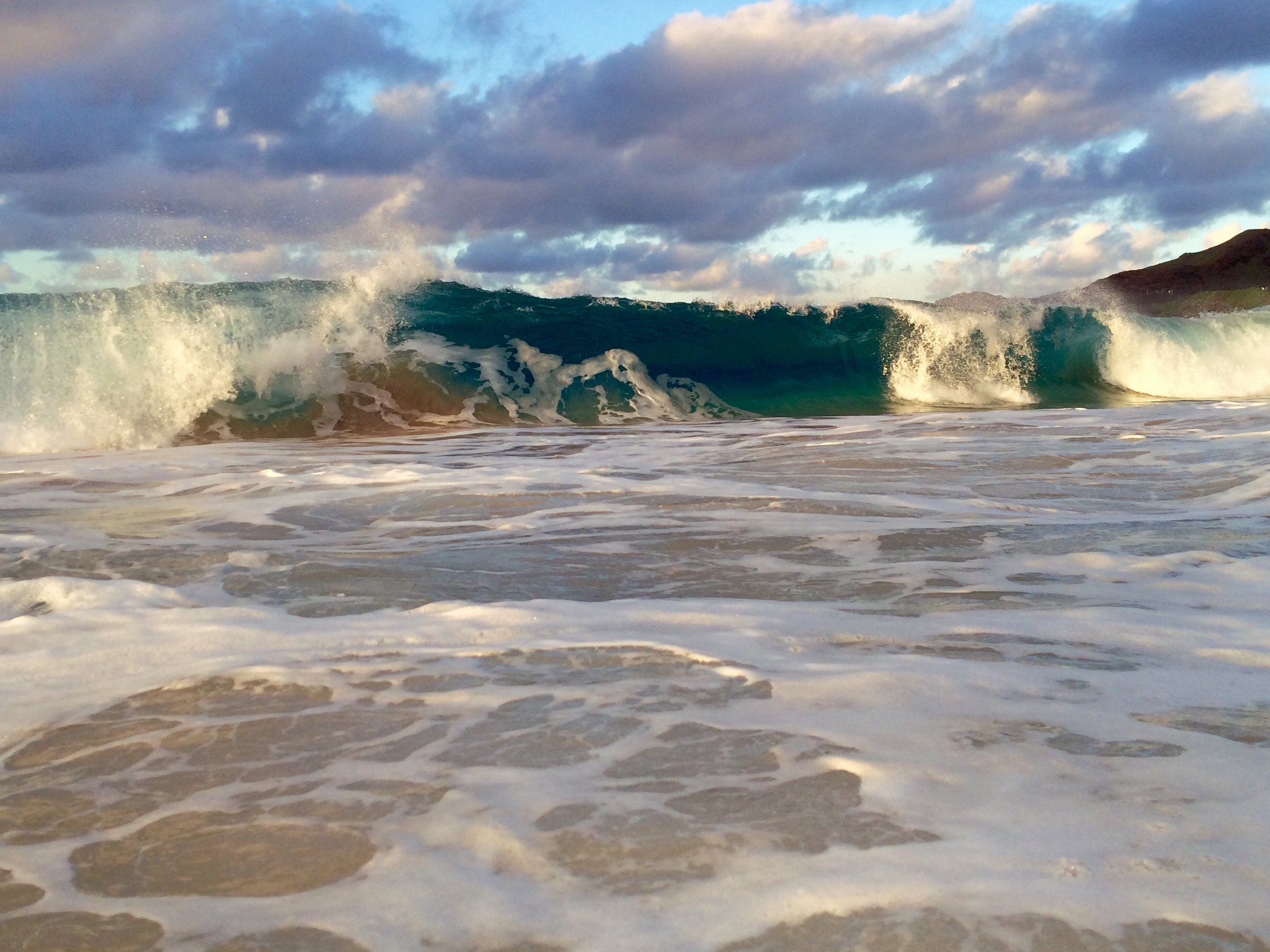A breathtaking photograph captures the untamed beauty of Big Surf. The scene is dominated by massive teal blue waves rolling in, their crests adorned with cascading white foam that stretches all the way up to the golden sand beneath our feet. As the tide advances, delicate wisps of foam travel across the beach, creating a mesmerizing pattern on the shore. In the background, a vast blue sky is dotted with large, rolled clouds. These clouds, backlit by the Sun, have their upper edges illuminated, while their bodies remain a deep, thunderous blue, scattered yet striking. The entire setting is drenched in serene sunlight, contributing to the tranquil yet powerful ambiance of the scene. There are no signs of human presence or man-made structures, emphasizing the pure, unspoiled nature of the landscape. To the right, a rugged brown mountain extends out of the frame, adding a touch of earthy grandeur to the picturesque view. The image is a vivid portrayal of Big Surf on a bright, sunny day, capturing the essence of untamed coastal beauty.